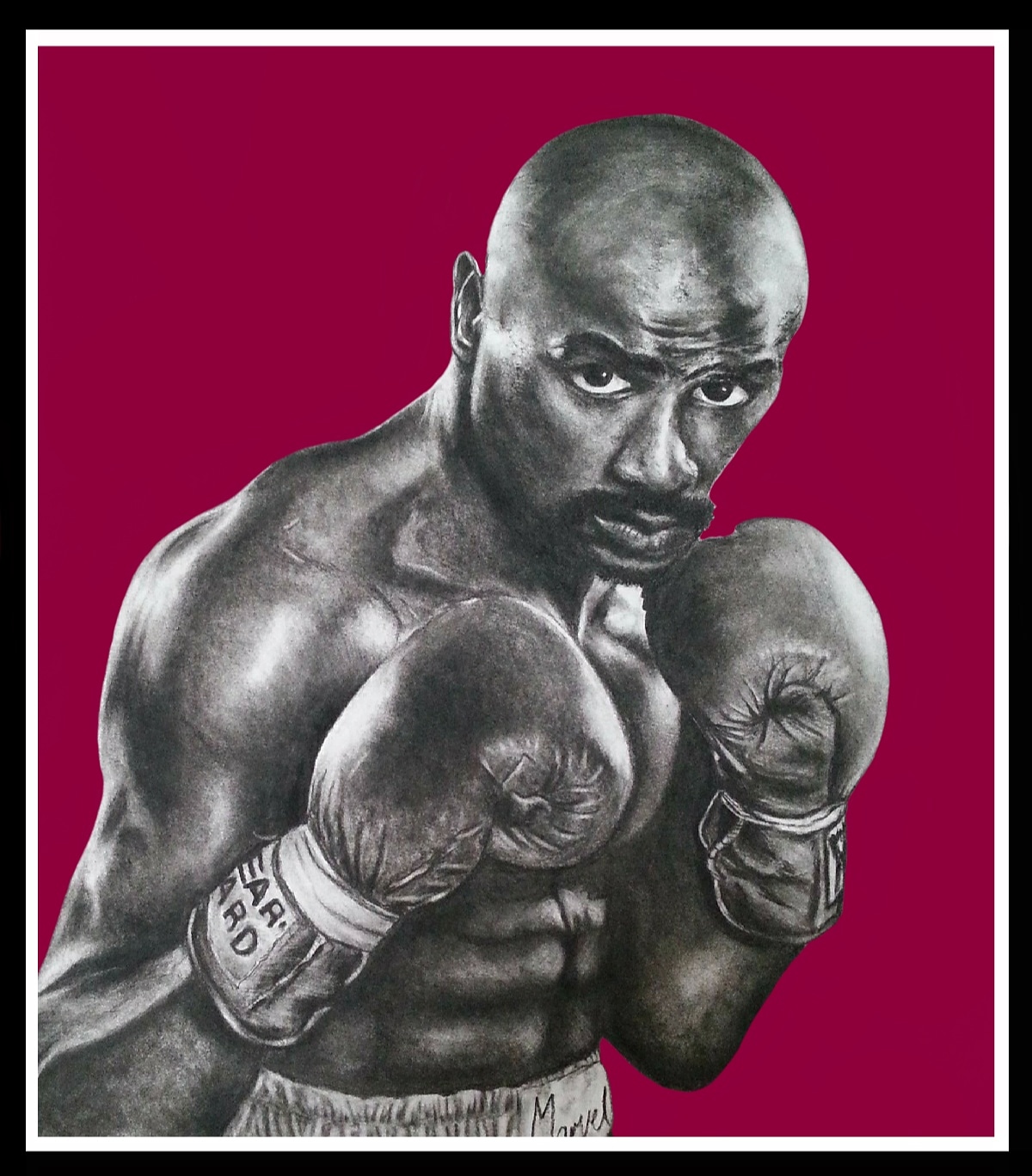The poster features a meticulously shaded, black-and-white pencil drawing of the iconic boxer, Marvelous Marvin Hagler, set against a rich maroon red backdrop. The image is bordered first by a black frame and then a crisp white border. Marvin Hagler, an African American with a bald head and a prominent mustache, stands poised in a classic boxer's stance, slightly turned to the right and gazing directly ahead. His muscular physique is highlighted, showcasing pronounced abs and shoulders. He dons boxing trunks inscribed with "Marvel" at the center, and both his hands are gloved and raised, ready for combat. The artwork captures the raw intensity and power of the legendary boxer, emphasizing his readiness for the fight.